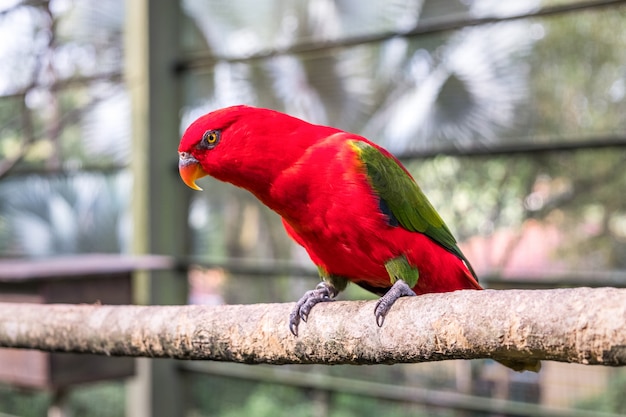In this detailed image, we see a vibrant, dark red parrot, predominantly red with striking dark green wings and legs accented by a small amount of yellow near the shoulders. The parrot is perched on a thick, horizontally suspended branch in the bottom third of the picture, facing left. The bird has an orange beak with a yellow tinge, orange eyes, and charcoal-colored feet. This scene appears to be set within a zoo or a conservation area, as indicated by the surrounding enclosure. In the background, there is a blurred but visible wooden framework with metal bands or thick black wires, likely supporting a glass or plastic barrier. Outside the enclosure, trees and foliage are discernible, adding to the naturalistic setting. To the left of the frame inside the enclosure, there is a wooden platform, possibly for a handler or for the bird's shelter.